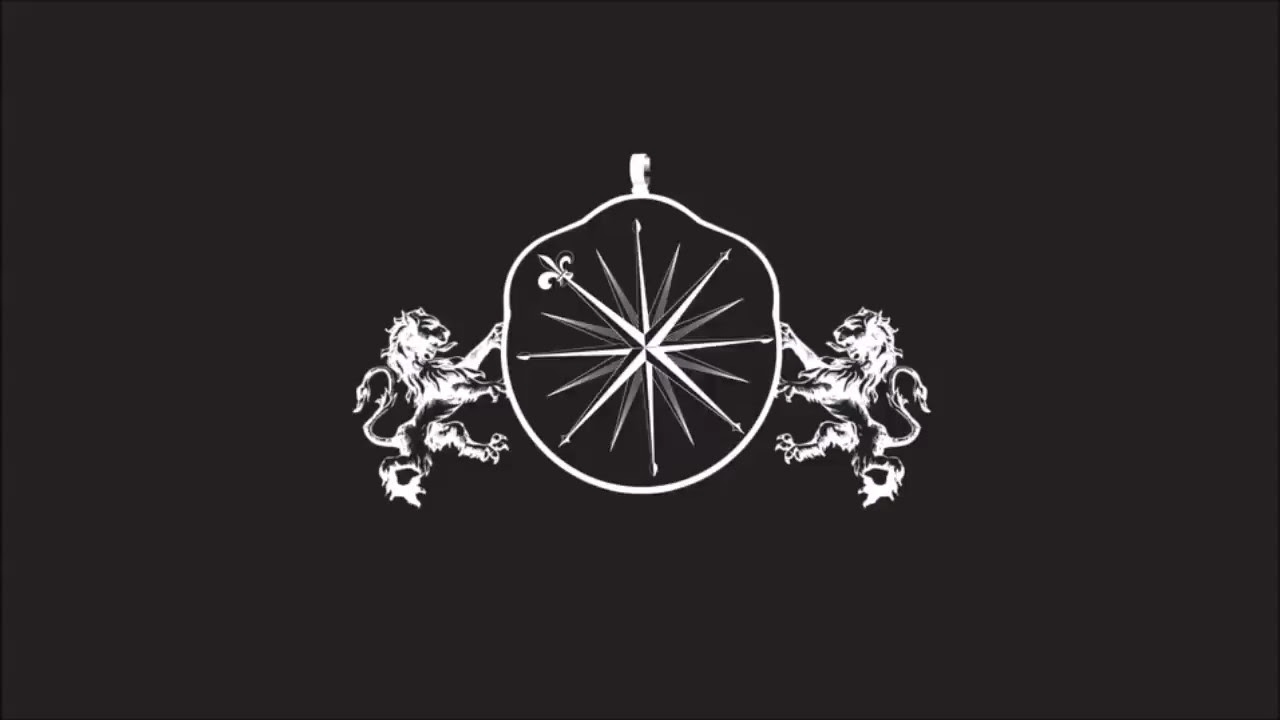The image depicts a detailed emblem set against a stark black background. Central to the emblem is a shield, acorn-shaped with a slightly irregular form, rendered in white. At its core, the shield features a prominent, star-like compass design with spikes radiating outward. Notably, one spike extends towards the top left, flaring out suggestively, and there is a chain hole or hook atop the shield, resembling a locket.

Flanking the shield are two identical, stylized lions, mirror images of one another, depicted in intricate detail with long, shaggy manes and sharp claws. Each lion is poised on its hind legs, with one paw from each lion gripping the sides of the shield. The lions, though white, appear strikingly against the black background, enhancing their royal and powerful demeanor. The overall effect is both dramatic and heraldic, with a sense of motion as the lions seem to leap towards the shield, emphasizing the emblem's dynamic composition.